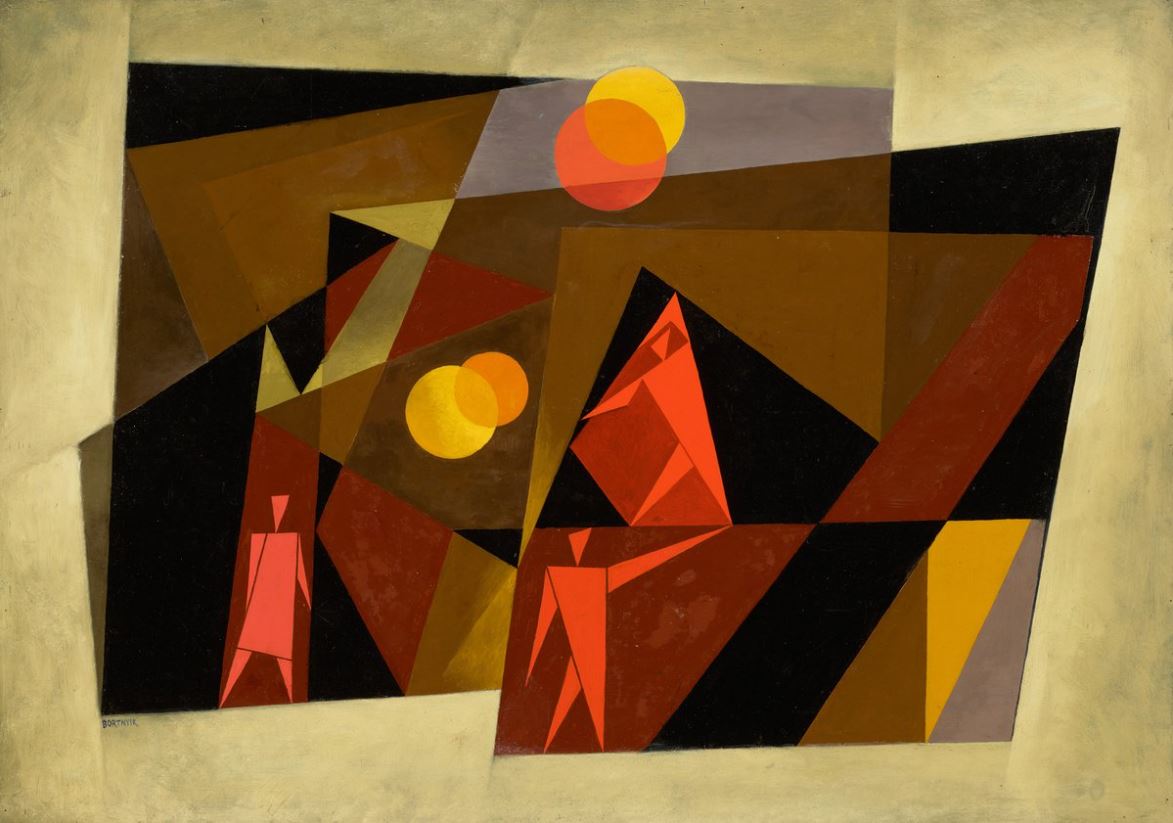This abstract painting, set on the back of old paper, is signed by the artist Sandor Bortniak in the bottom left corner. The composition features a beige background with accent shades of green and is rich in a variety of colors including black, brown, red, orange, yellow, light blue, and maroon. Dominating the painting are overlapping circles at the top that mimic a sunset, with an orange circle slightly larger than the yellow one behind it. The central image is a combination of various shapes and patterns, primarily circles and triangles. Within the red and maroon triangular forms are simplistic, orange stick-figure men with triangular bodies, arms, heads, and legs, depicted three times in different poses. These figures are placed toward the bottom center, just above in a profile view, and on the lower left. The overall artistic style is a modern, figurative abstraction, echoing influences that became popular in the 1940s and 50s. The painting’s title is "Bortniak Sande Paritz Langzai."